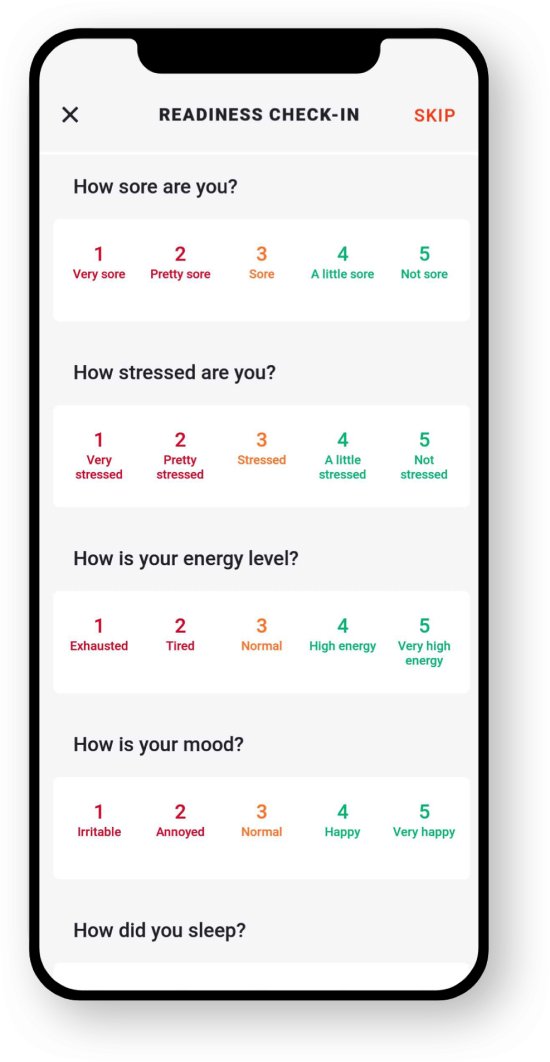The image is a detailed screenshot of a digital survey interface designed for assessing readiness and personal metrics. The screen is bordered by a thick black frame. Along the top, a black tab extends from about an inch from the left side, spanning across to an inch from the right side before returning to the border. Within this tab, bold black letters read "READINESS CHECK-IN", with a red "SKIP" option on the right side and a black "X" on the left.

Below this tab is a narrow white border followed by an inch-thick gray section and another inch of white space. Embedded in the gray section, black text poses the question, "How sore are you?" followed by five response options evenly spaced from left to right. The options are:
- Very Sore (1) in purple
- Pretty Sore (2) in purple
- Sore (3) in orange
- A Little Sore (4) in teal
- Not Sore (5) in teal

Beneath this question, another gray section appears with the query, "How stressed are you?" using the same color coding for options:
- Very Stressed (1)
- Pretty Stressed (2)
- Stressed (3)
- A Little Stressed (4)
- Not Stressed (5)

Following this, another gray section asks, "How's your energy level?" again with the same color-coded scale:
- Exhausted (1)
- Tired (2)
- Normal (3)
- High Energy (4)
- Very High Energy (5)

Next, the gray section presents the question, "How is your mood?" with similar color codes:
- Irritable (1)
- Annoyed (2)
- Normal (3)
- Happy (4)
- Very Happy (5)

Finally, the bottom part of the image includes a gray section asking, "How did you sleep?" though, only the top edge of the corresponding white box is visible, suggesting it follows a similar structure to the previous sections. 

Overall, the interface is methodically organized with consistent color schemes and structured questioning to facilitate a comprehensive readiness check-in.